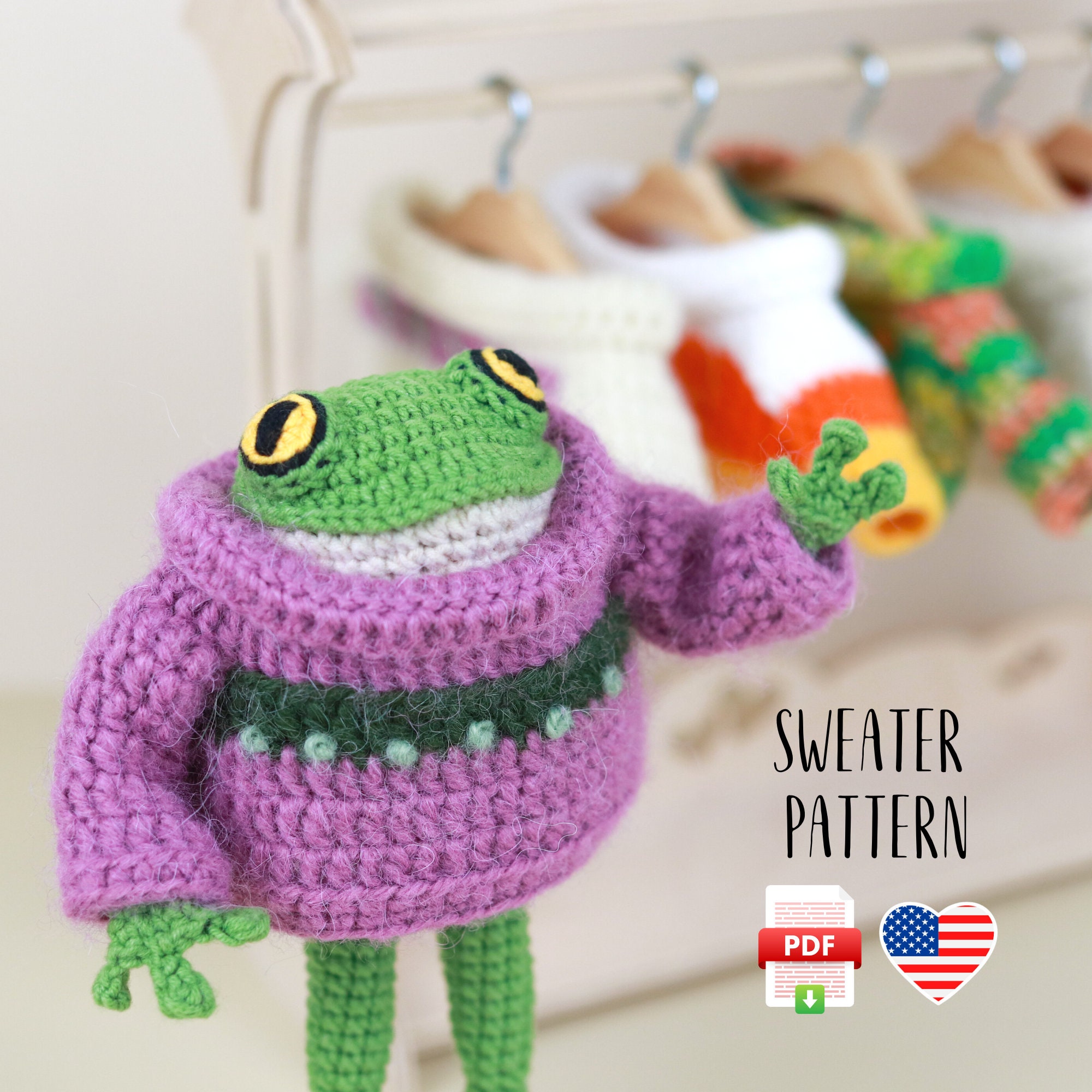This detailed photograph features an intricately crocheted or knitted green frog with vibrant yellow eyes, a white belly, and three-fingered hands, standing on its green legs. The frog is wearing a striking purple turtleneck sweater, adorned with a central green stripe embellished with delicate blue dots. It appears to be waving with its right arm raised. The background reveals an array of similar miniature sweaters on tiny hangers, suggesting a wardrobe for the frog. Most of the background is an off-white or pale grey, drawing focus to the vibrant colors of the frog and its sweater. At the bottom right corner of the image, the text reads "Sweater Pattern," alongside a PDF download symbol and a heart containing the American flag, indicating the pattern's availability and American origin. This image likely serves as an advertisement or social media post for a crochet or knitting pattern download.